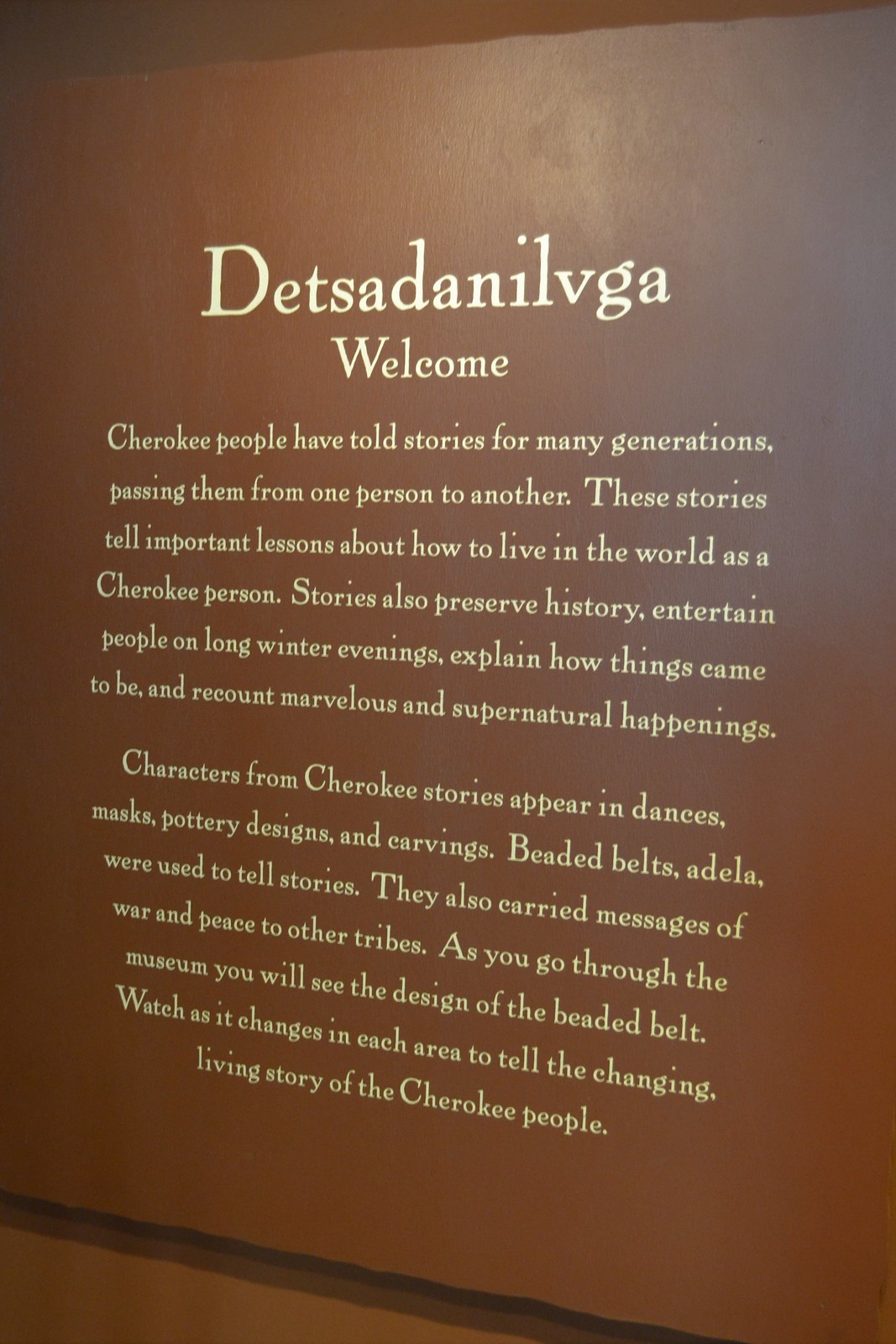This photograph showcases a brown plaque with gold and white text, prominently featuring the Cherokee word "Dets-ta-da-nee-vil" or "Detsa Danlivka," which translates to "welcome." The plaque provides an insightful explanation about the significance of storytelling in Cherokee culture. It details how Cherokee people have passed stories from generation to generation, preserving history, teaching important life lessons, providing entertainment during long winter evenings, explaining natural phenomena, and recounting marvelous and supernatural events. The stories also manifest in various art forms such as dances, masks, pottery designs, and carvings. Additionally, the plaque highlights the use of beaded belts, or "adela," which were not only used to tell stories but also to carry messages of war and peace between tribes. As visitors proceed through the museum, they are encouraged to observe the changing designs of the beaded belts, which reflect the dynamic and evolving narrative of the Cherokee people.